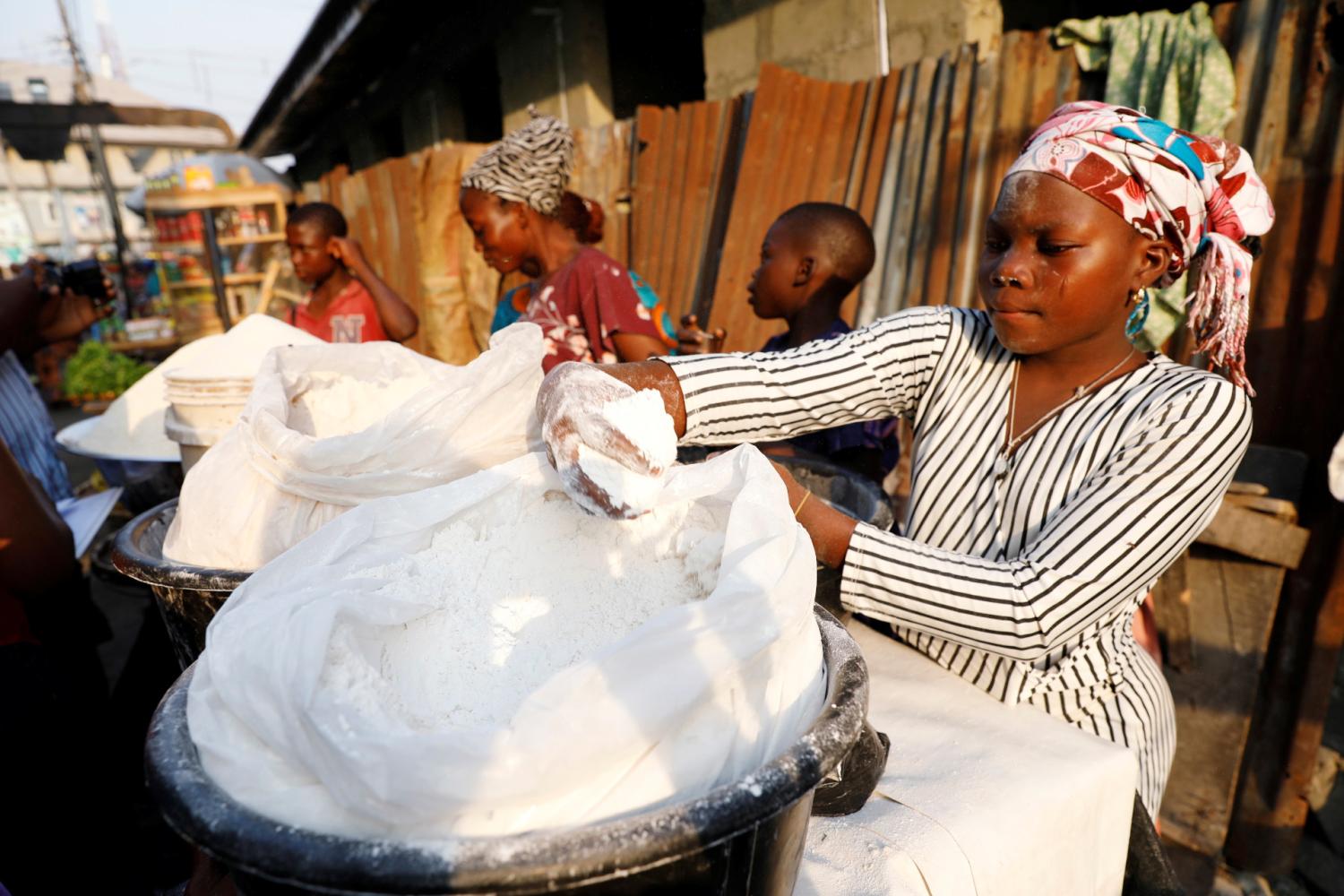The image captures a vibrant and busy scene in what appears to be a tropical outdoor market or work area, possibly in an African or Caribbean country. The photograph is in full color, horizontal in format, depicting several individuals of African descent. 

In the foreground, a focused woman, dressed in a white and black striped shirt and a multicolored headscarf, is prominently featured as she meticulously scoops a white powdery substance, possibly flour, from a bag lined inside a large plastic trash can or laundry tub. This gives a strong sense of her being engaged in a significant task. 

To her left, another woman and a young boy appear to be conversing while engaged in a similar activity, indicating a collaborative effort. Even further to the left, another young boy participates in the same task. This entire group is working amidst bright sunshine, suggestive of a tropical locale.

Behind them stands a seven-foot sheet metal or wooden fence, adding a boundary to their work area, with possibly a building in the background. All individuals are dressed in colorful, likely culturally significant clothing, including ornate headscarves for the women. The scene below them features dark gray or black containers, which could be laundry tubs, with traces of foam or soap spillage, blending with the white powder around, adding layers of texture to the daily chore atmosphere.